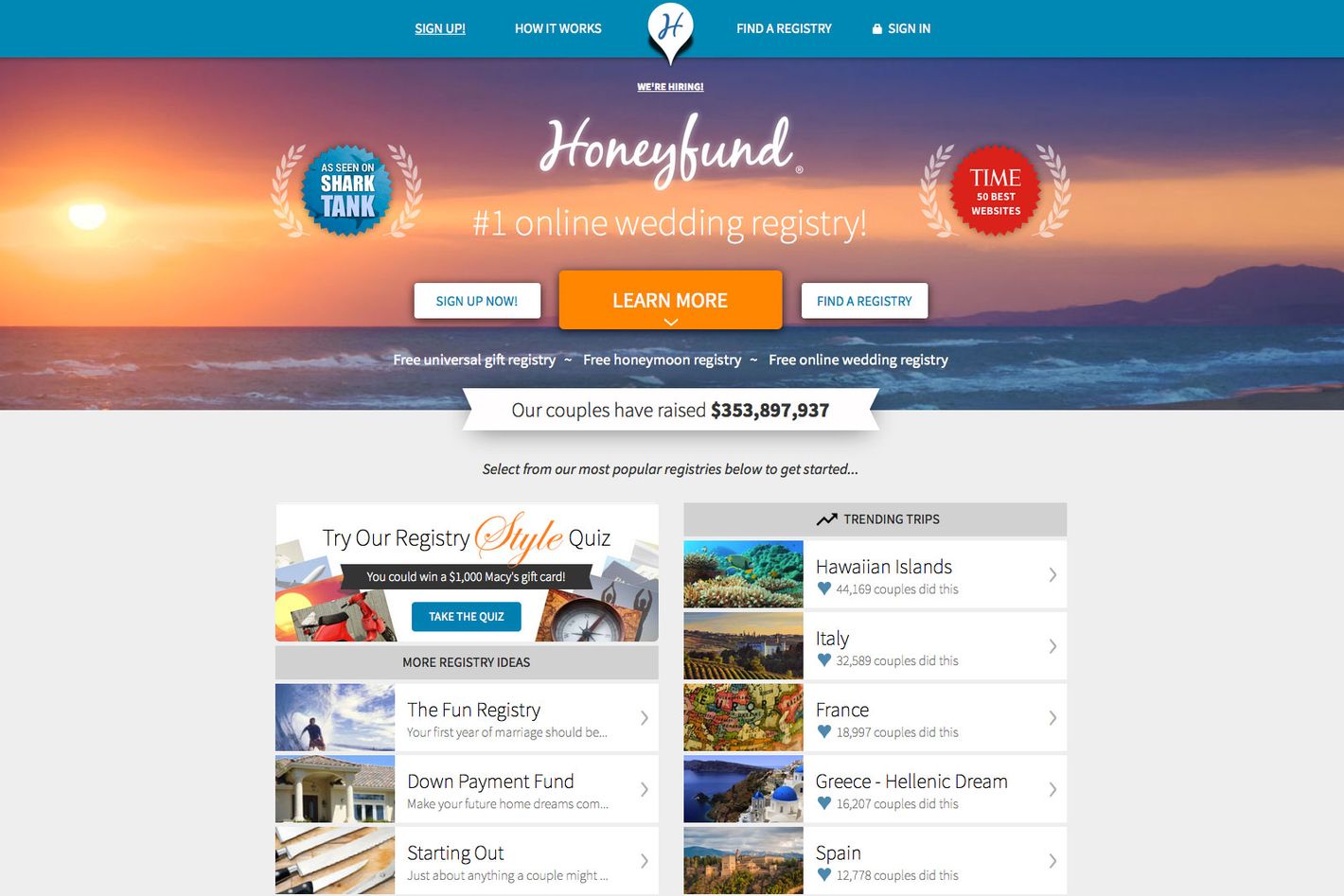This screenshot captures a webpage from an unknown website viewed on a computer. At the top of the page, there's a blue border with various options and buttons displayed in white text. These include a "Sign Up" button, a "How It Works" button, and a logo resembling an upside-down drop with the letter "H" in blue against the white background of the drop. Additionally, there are "Find a Registry" and "Sign In" buttons.

The page prominently features the name "TinyFund" and touts itself as the "#1 Online Wedding Registry." The main call-to-action encourages visitors to "Sign Up Now." Further down, the site offers more functionalities like "Find a Registry." 

The main content showcases trending honeymoon trips with destinations such as Hawaiian Islands, Italy, France, Greece, and Spain. Accompanying the list are visually appealing images that invite users to explore further. Also present on the page is an interactive quiz intended for user engagement.